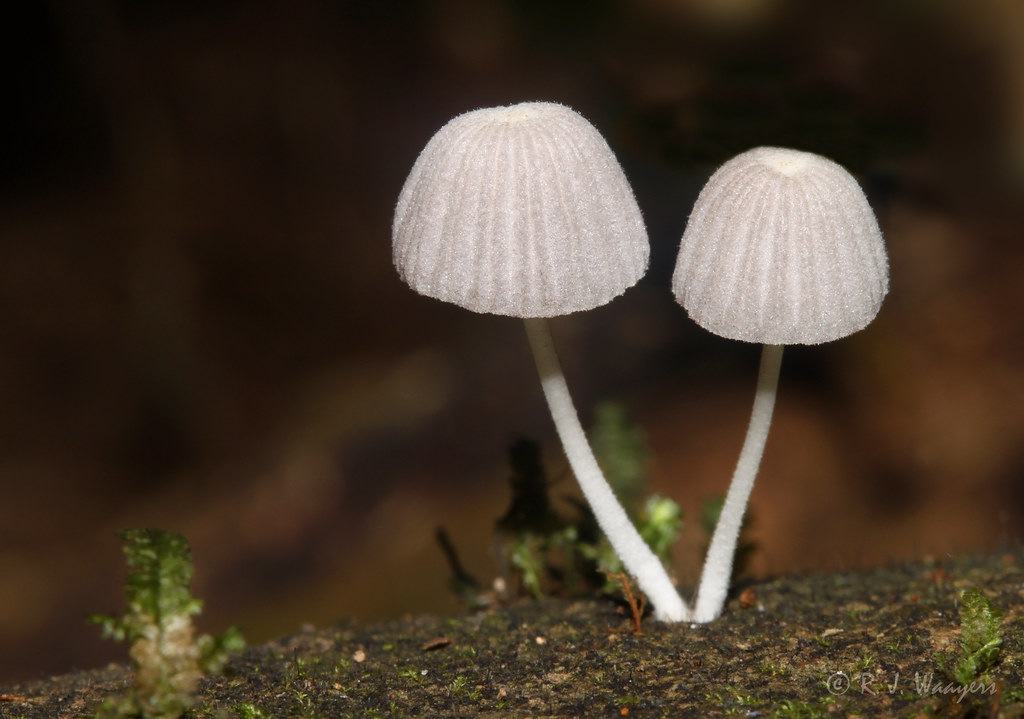This close-up photograph showcases two tiny, delicate mushrooms emerging from dark, textural soil. Both mushrooms, adorned with pristine white stems and bell-shaped caps, rise from the same point but curve outward in opposite directions. The mushroom on the left is slightly taller and larger compared to its companion. Surrounding the fungi, hints of vibrant green moss add a touch of color and life to the earthy scene. The background features a blend of black and brown hues, giving it a rich and textured appearance. In the lower right-hand corner of the image, there is a copyright watermark that reads "C.R.J. Wagner."